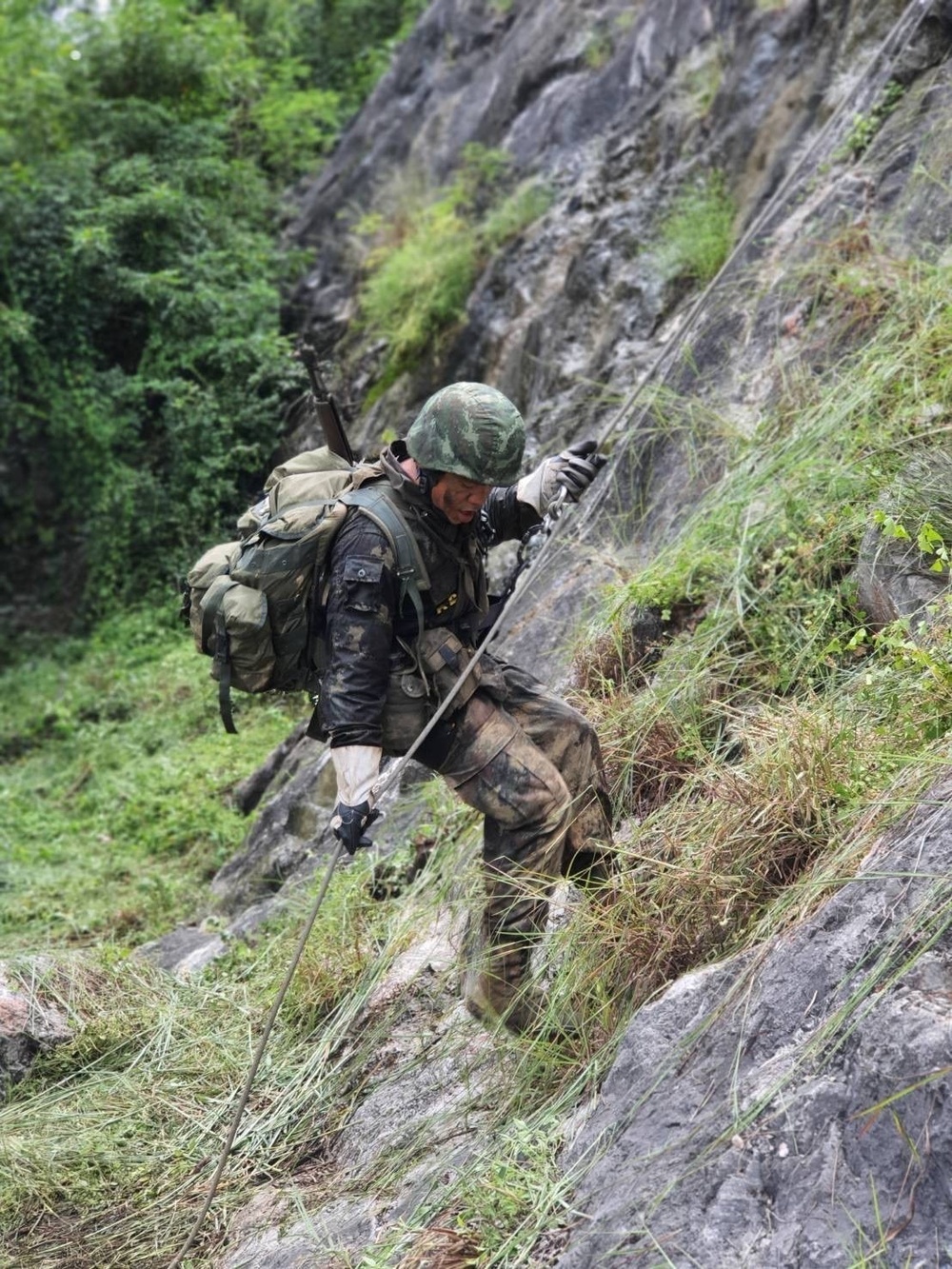An army soldier, who appears to be of Asian descent, is rappelling down a sheer, rocky mountainside. The soldier is fully equipped in his military gear, including a green camouflage uniform, a camouflaged helmet, and black gloves. A large green backpack is strapped to his back, with a rifle partially protruding from it. He is secured with ropes and braces, navigating his descent on a thick white rope. The rocky terrain he scales is a mix of grayish-brown stone with patches of green foliage and yellow, straw-like grass. In the background, a lush scene of vibrant green trees and dense foliage indicates the hillside extends into a forest. The soldier, gazing downward as he maneuvers, is adorned in navy green camouflage, which seamlessly blends with the natural environment.